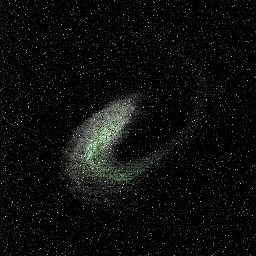The image depicts a starry sky set against a small, square black background, densely populated with numerous white specks representing stars. These stars are scattered throughout, yet more densely clustered towards the center, where they form a concentrated, swirly sea-like pattern that tilts counterclockwise. This central feature, reminiscent of a nebula or galaxy, appears almost like a swoosh of white amidst the predominantly black backdrop. The density of stars diminishes towards the bottom, elongating the appearance of the sea-like formation. Together, these elements create a striking visual of a night sky teeming with stars, highlighted by the swirling concentration at its core.